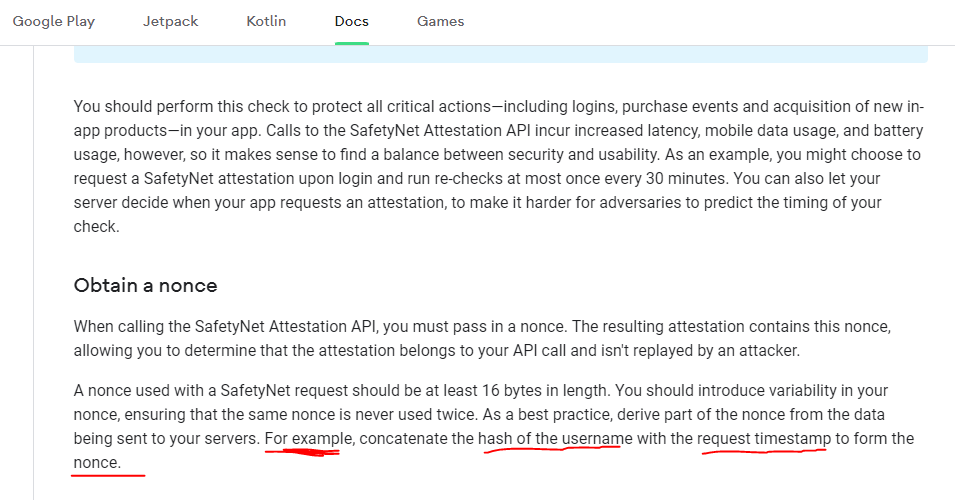The screen displays the Google Play console with a clean white background and dark text. At the top, a navigation menu offers several options: "Google Play" in the corner, followed by "Jetpack," "Kotlin," "Docs," and "Games." The "Docs" option is underlined in green, indicating that it is the currently active section.

The main body text begins with a guideline: "You should perform this check to protect all critical actions, including logins, purchase events, and acquisition of new in-app products in your app." Below this, a new section starts with the header "Obtain Nonce." The first line reads, "When calling the Safety Net Attestation API, you must pass in a nonce."

The text includes detailed instructions and explanations, with certain phrases underlined in red for emphasis. For example, in the sentence that follows, the phrases "hash of the username" and "request timestamp" are distinctly marked. The text suggests, "Concatenate the hash of the username with the request timestamp on the nonce," providing specific examples and best practices for implementing security measures.